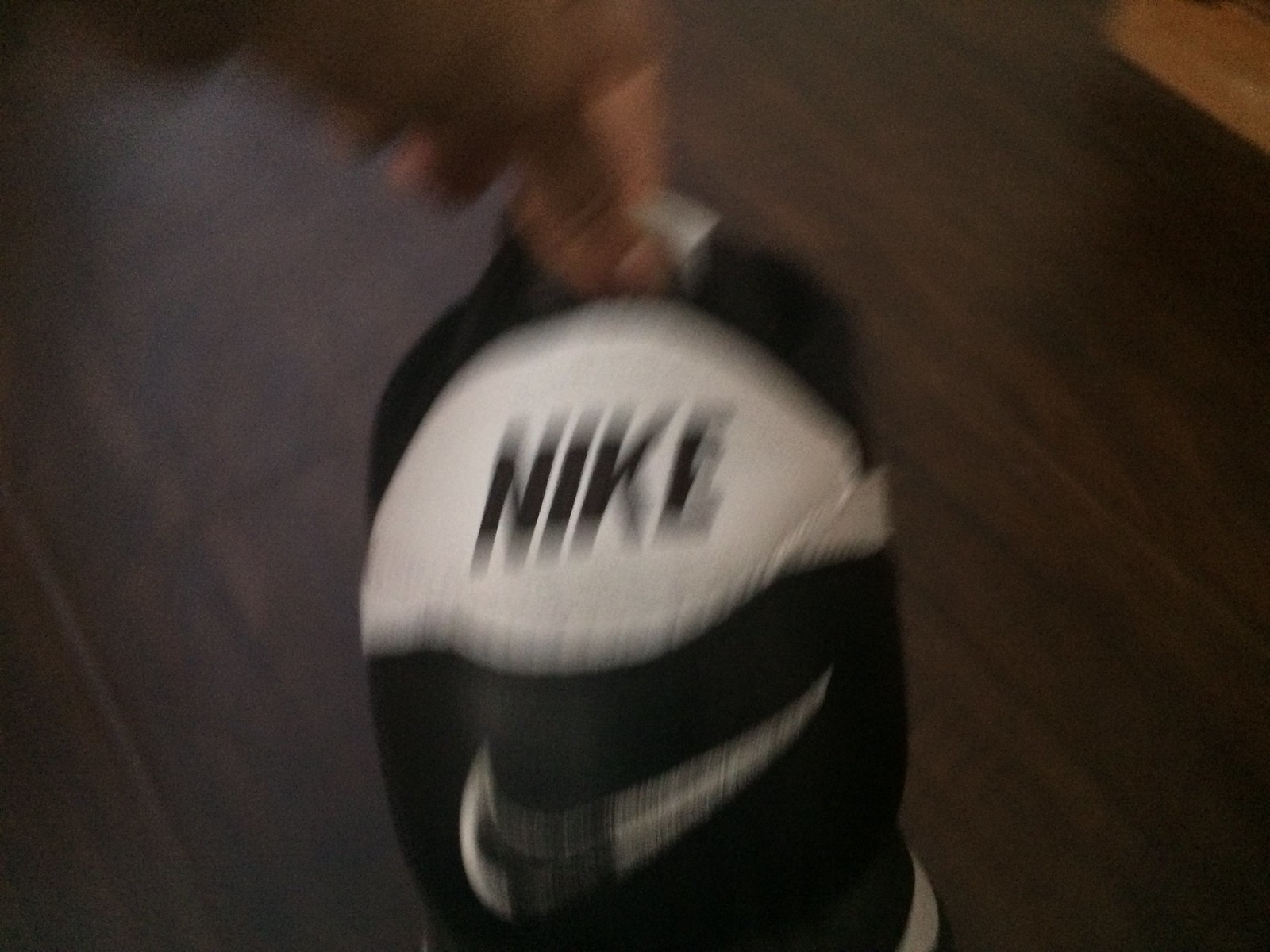This is a very blurry image featuring a person of darker complexion, possibly a Black individual, attempting to lift a Nike bag off brown wooden flooring. The Nike bag is prominently white with black lettering spelling "NIKE" in the center, and features the iconic Nike swoosh logo, which is mostly white with some black accents. The wall in the background has an orangish tinge.